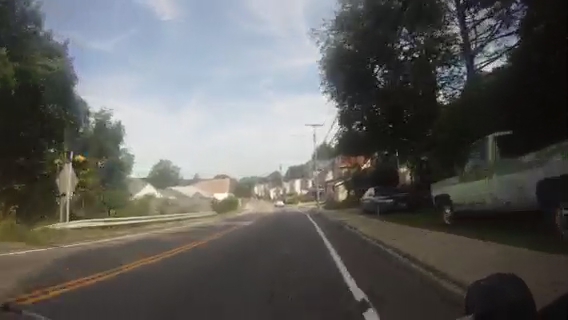This photograph, likely taken from a moving vehicle or a bike, captures an outdoor scene along a two-lane paved road with gray pavement, distinguished by white lines on the edges and a double yellow line in the center. The image features a blue sky with wispy white clouds stretching above the scene. To the right, a white truck with green on top and a sedan are parked just past a white sidewalk, alongside trees that extend to the upper right corner of the image. On the left, more trees line the road alongside a rail, adding to the suburban ambiance. Above, electrical power lines can be seen, leading towards a cluster of four or five white and brown homes in the distance. Despite its blurry and slightly pixelated appearance, reminiscent of a high-end video game, the photorealistic quality suggests it is indeed a photograph.